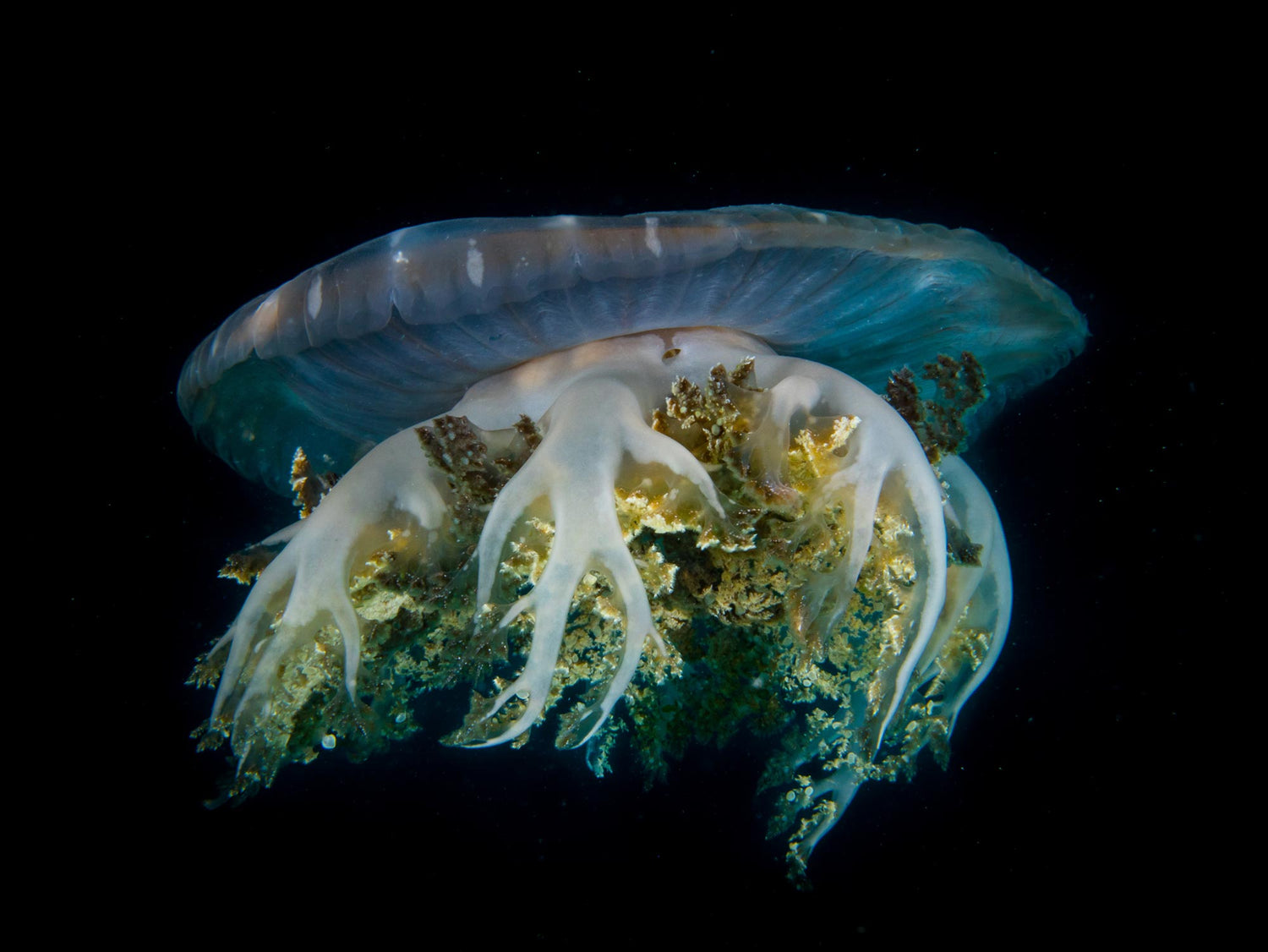The image features a central, otherworldly figure resembling a jellyfish floating against a stark black background, giving an impression of deep-sea mystery or perhaps a night sky with stars. At the top, there is a blue, translucent dome-like shape with subtle red hues underneath its surface, possibly hinting at a luminescent sea creature such as a Portuguese man-of-war. From the bottom of this blue dome, gnarled, white tentacle-like branches extend downward, enveloping an array of plant-like structures beneath them. These plant forms, which suggest the appearance of algae or leafy vegetation, showcase a mix of gold, brown, and deep green colors. The white tendrils almost appear to be frosting, adding to the surreal and possibly digitally altered aesthetic of the scene. This intriguing mix of marine biology and fantastical elements creates a captivating and somewhat mysterious image, blending the natural with the imaginative.